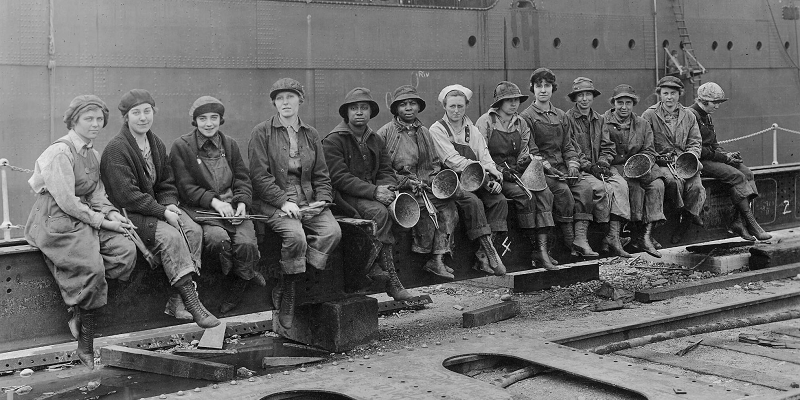This is a vintage black and white photograph, likely from the early 1900s, depicting a group of approximately 13 women working at a construction site, possibly related to a submarine or ship. The women are seated on a large metal I-beam, which features visible numbers. Behind them is a structure resembling a ship or submarine, identifiable by numerous portholes dotting its side. The women, dressed in hats and work overalls with boots, appear weary and dirty, likely indicating the hard labor they've been engaged in. Some of them are holding bowls, tools such as clamps or pliers, and conical-shaped metal devices. Debris from their work is scattered on the ground in front of them. All but one of the women are looking towards the camera, posing for the photograph.